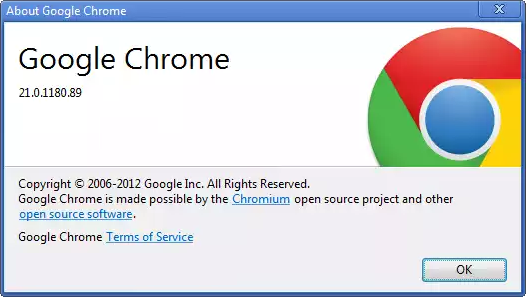This image displays an older "About Google Chrome" pop-up window, illustrating the browser's version information and details. The version number is 21.0.1180.89, highlighting that this iteration of Google Chrome was from the years spanning 2006 to 2012, as indicated by the accompanying copyright ©2006-2012 by Google Inc., All Rights Reserved. The pop-up credits the Chromium Open Source Project along with other open-source software as instrumental in Chrome's development. 

Central to the pop-up is Google Chrome's iconic circular logo, divided into segments of red, green, yellow, and blue, providing an immediate visual association with the browser. The upper right-hand corner of the window features an "X" button for closing the pop-up, signifying standard UI design of the time. 

Within the textual content, several hyperlinks are embedded: "Chromium," "open source software," and "Google Chrome Terms of Service." These links are distinguishable by their blue, underscored text, although the exact destinations are not visible in the image. 

A prominent OK button is situated at the bottom of the window, inviting users to acknowledge and close the pop-up. This specific type of pop-up window was commonly accessed through Chrome's Help menu under the "About" section, enabling users to verify their browser version for updates or troubleshooting purposes.